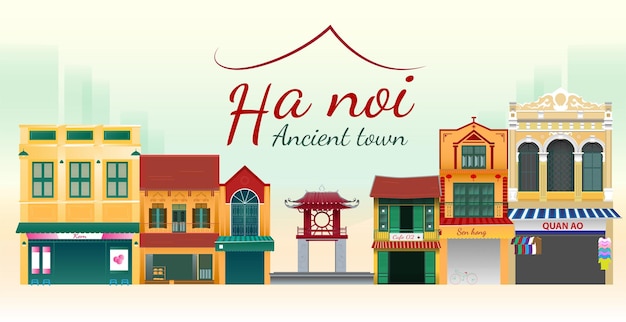The image depicts a vibrant and colorful cartoonized banner likely intended for a website, showcasing an ancient town scene from Hanoi. The top center of the banner prominently displays the text "Hanoi" in red font, with "ancient town" written directly below it in black font. A distinctive V-shaped line arches above the word "Hanoi." The street scene features an array of vividly colored buildings lined up as you might find in a bustling cityscape. These include a yellow building, a red building, an orange and red building, and in the middle stands a traditional Chinese shrine highlighted in red with gray pillars. Further in the background are additional green, orange, and beige buildings, with the beige one displaying a shop sign "Quan Ao" and an eye-catching pink heart in one of its displays. The vibrant storefronts below appear to double as both shops with bright awnings and colorful posters, and residential apartments above. Beyond these structures, the background shows a hazy sky with contrasting skyscrapers on both sides, set against a primarily white backdrop that accentuates the lively and vivid colors of the buildings in the foreground.